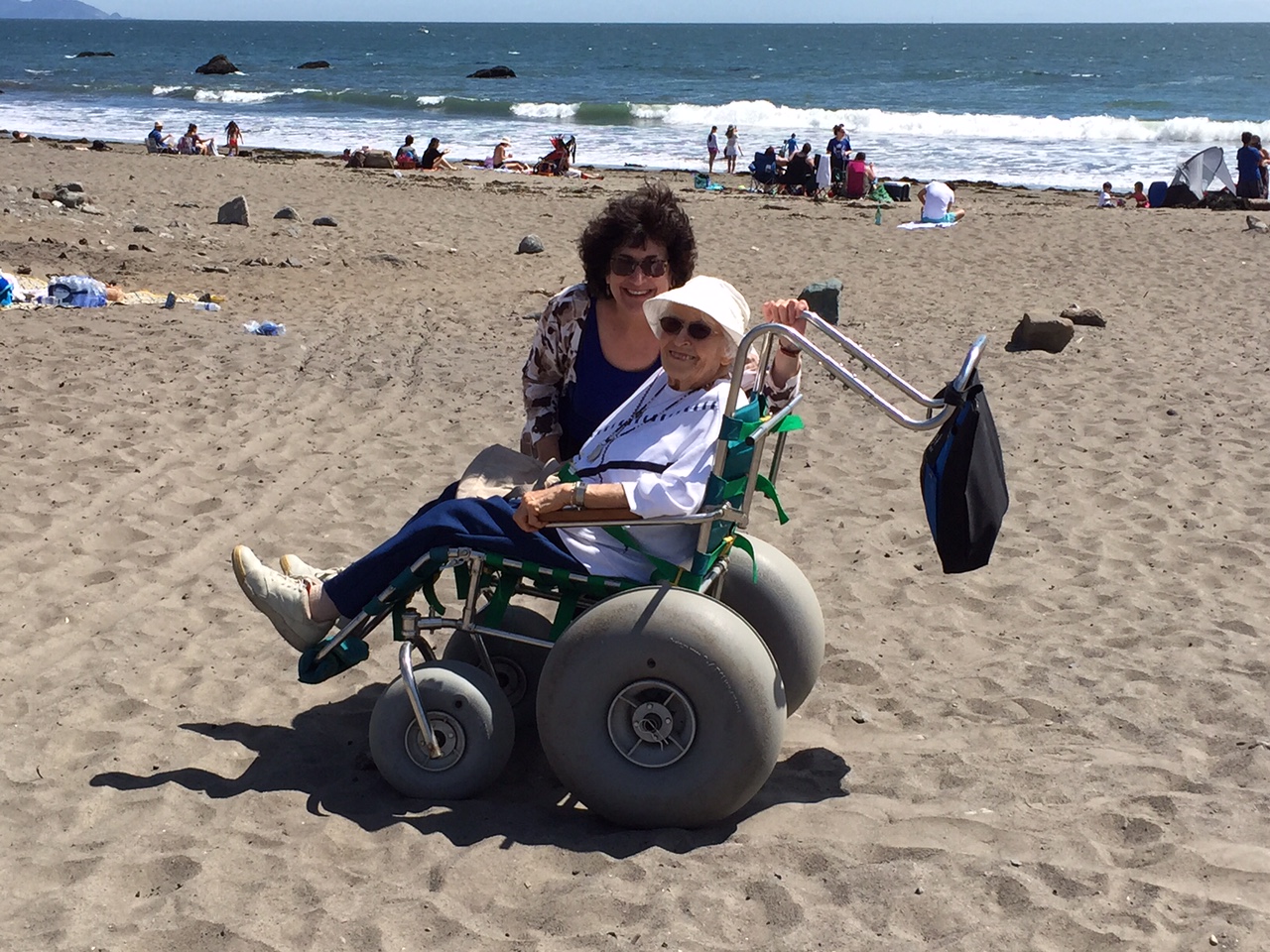In this detailed color photograph, set in a lively beach scene, an elderly woman sits in a specialized electric wheelchair designed for sandy terrain, featuring oversized, inflated tires, particularly massive at the back. The woman, smiling warmly, is adorned in a beige sun hat, sunglasses, a white t-shirt layered with a sweatshirt, blue pants, and beige footwear. Attached to the back of the wheelchair is a black bag, possibly her purse. Beside her, a younger woman, potentially her daughter, also smiles into the camera. She has dark, puffy hair, wears sunglasses, a black tank top, a blue shirt, and a white and brown overshirt. The beach stretches out behind them, showcasing the ocean waves, a clear sky, and numerous beachgoers scattered across the frame, lounging, chatting, and observing the sea. To the left of the wheelchair, a person is lying on the sand. The image captures this serene yet vibrant beach moment with photorealistic detail, highlighting both the individuals and the expansive natural backdrop.